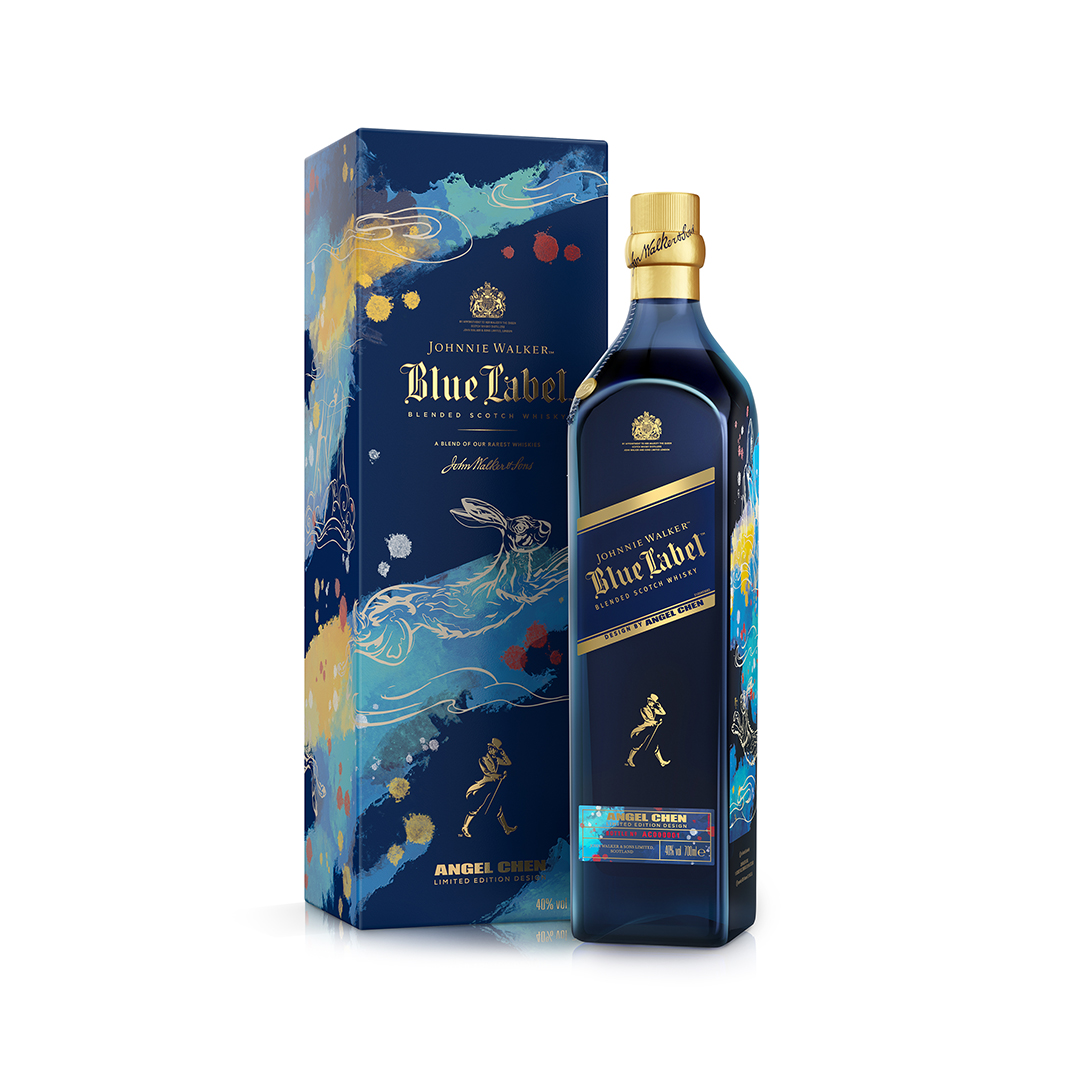This photograph showcases a regal product shot of Johnny Walker Blue Label, a premium blended scotch whiskey. The centerpiece of the image is the dark blue, slightly translucent bottle, adorned with the iconic gold-capped top and the classic Johnny Walker label featuring the distinguished man in a top hat, coat, boots, and cane. The label prominently displays "Johnny Walker Blue Label" diagonally, with the name "Angel Chen" inscribed below. Complementing the bottle, the accompanying navy blue box mirrors the bottle’s design with gold lettering and includes a striking blue rabbit motif. Both the bottle and the box are detailed with artistic splashes of sky blue and yellow, making for a visually captivating and luxurious presentation.